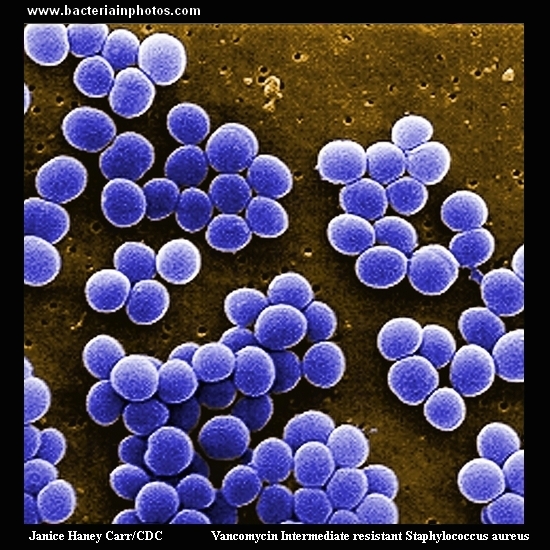This is a detailed microscopic photo of bacteria identified as Vancomycin Intermediate Resistant Staphylococcus aureus. The photo, which has a black border along its edges, prominently displays the website www.bacteriainphotos.com in white text at the top left. The bottom left corner specifies the photo credit to Janice Haney Carr from the CDC. The image captures the bacteria as clustered, blue spherical objects with white outlines. These spheres are positioned against a brown, porous background that features small holes. The bacterial clusters are predominantly in the middle bottom and top left sections of the image, while being sparser towards the top right and right side. The overall appearance of the bacteria closely resembles tightly packed clusters of grapes.